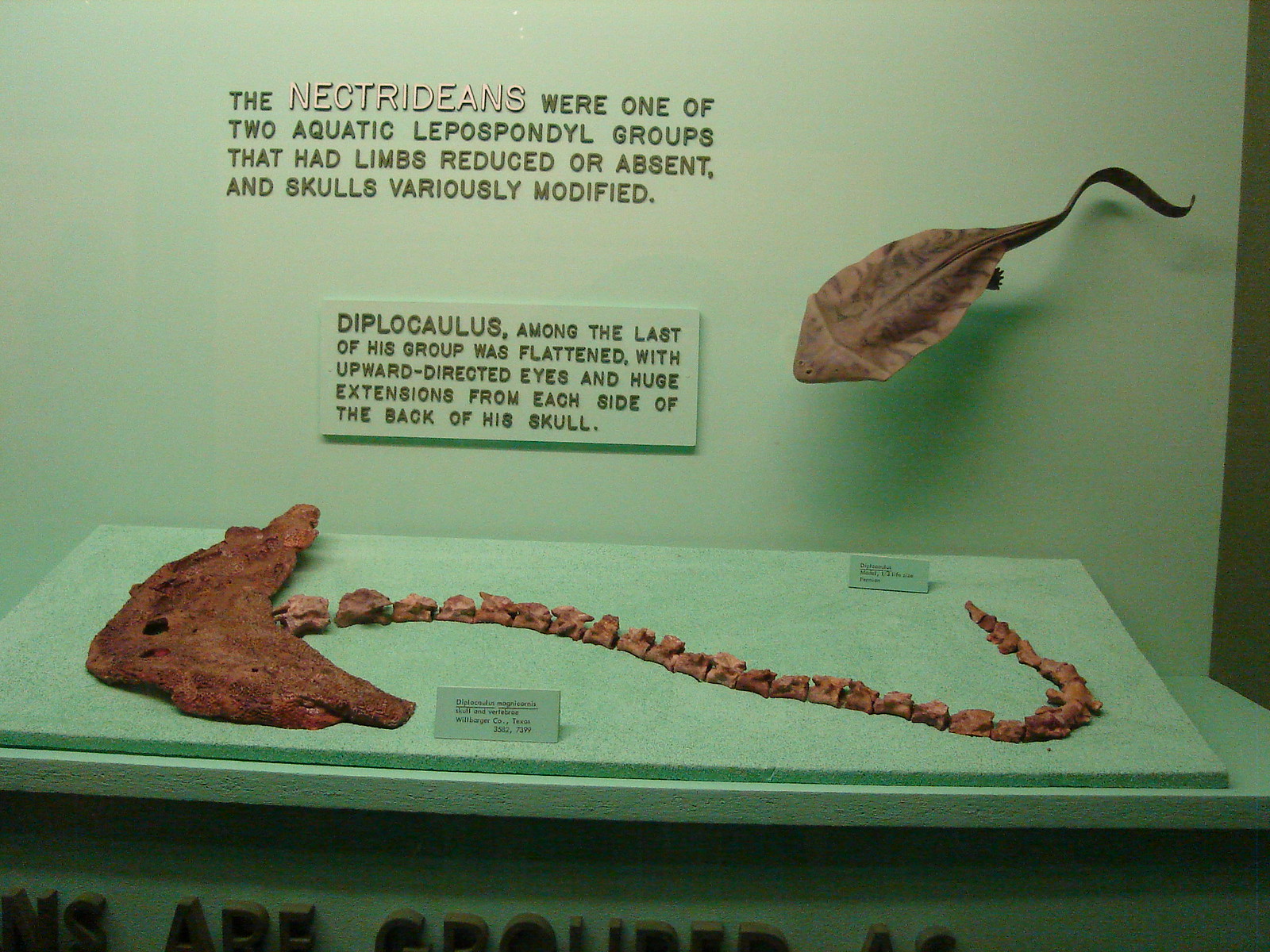This image is from what appears to be an animal museum or aquarium exhibit focused on ancient aquatic creatures. The display is encased in a green backdrop and features two main specimens: one laid on a platform and the other mounted on the wall. Both specimens seem to resemble stingrays or fish with significant skeletal features. 

The primary subject on the platform appears to be a fossil with a shape reminiscent of a stingray, possibly with an elongated tail. This specimen is accompanied by information cards, one positioned at the front and another at the back of the platform.

Mounted on the wall to the right, there's another fossil that looks tadpole-like, with physical characteristics suggesting adaptations for an aquatic environment. Both specimens are identified as Nectridians, which were one of the two aquatic Lepospondyl groups characterized by reduced or absent limbs and variously modified skulls.

The exhibit provides detailed information, stating: "The Nectridians were one of the two aquatic Lepospondyl groups that had limbs reduced or absent and skulls variously modified. Diplocolus, among the last of his group, was flattened with upward-directed eyes and huge extensions from each side of the back of his skull." The fossils exhibit these unique traits, underscoring their specialized adaptations for an aquatic life.